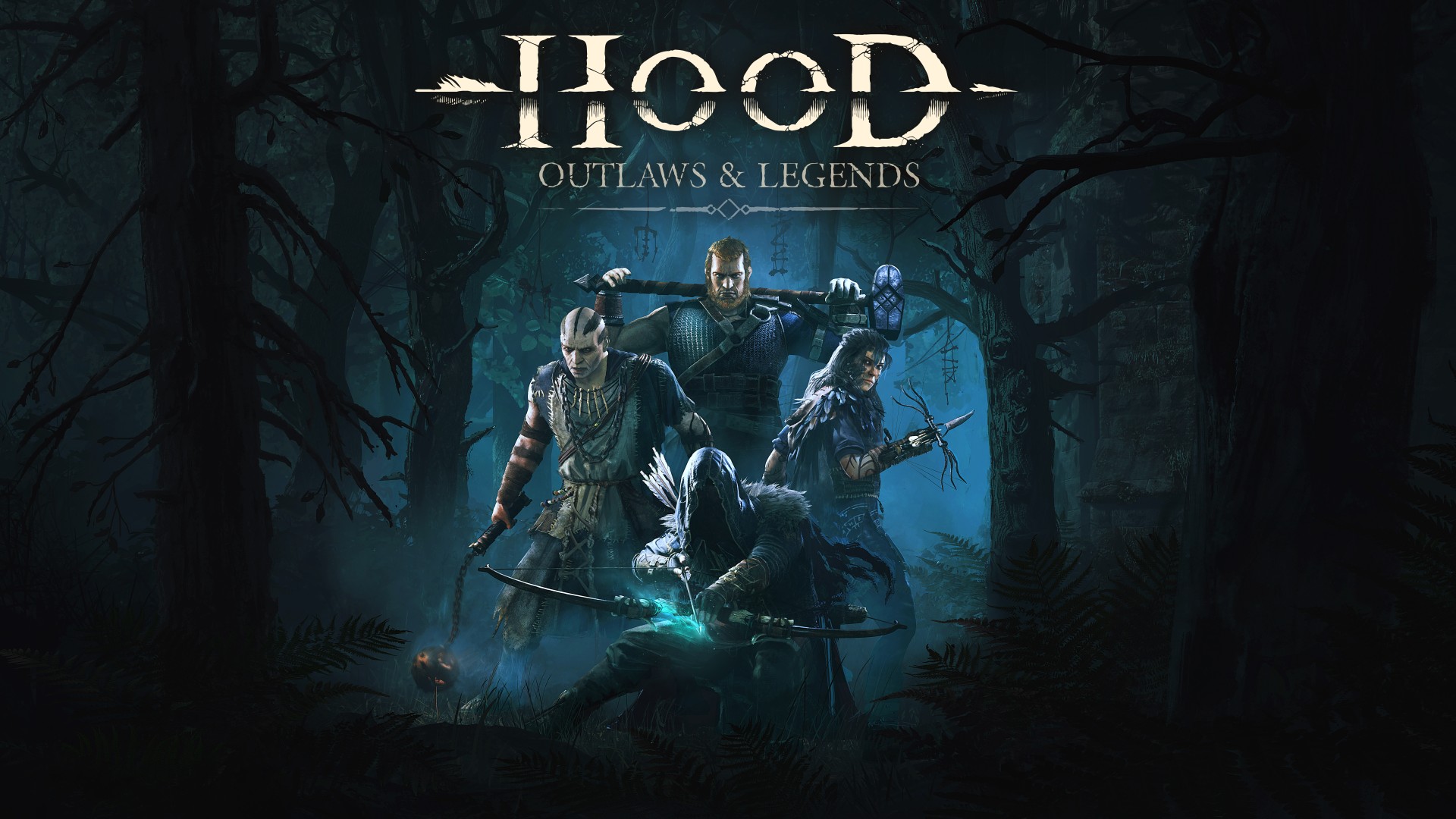This color image features a promotional scene, likely for a video game or movie titled "Hood: Outlaws and Legends," as indicated by the white text at the top of the image. The title "Hood" is notably pierced by an arrow, with the arrowhead emerging from the letter 'D' and the fletching visible near the 'H'. The setting is a dark, misty forest illuminated by an eerie blue light in the center, contrasting against the black, shadowy trees surrounding the characters.

In the foreground stands a hooded figure, face concealed in shadow, equipped with a large bow and a quiver of arrows, readying an arrow on the bowstring. To his left, a bald man with a pallid complexion, adorned with black makeup or tattoos, wields a spiked ball on a chain. This imposing figure is clad in dark, leather-like armor. On the right, another warrior with long black hair and an intense glare grips a knife. Behind them, a burly man with red ginger hair and beard, dressed in chain mail and crisscross black belts, hefts a massive hammer over his shoulders. The ensemble of characters is poised in readiness, set against the ominous and shadowy woodland backdrop.